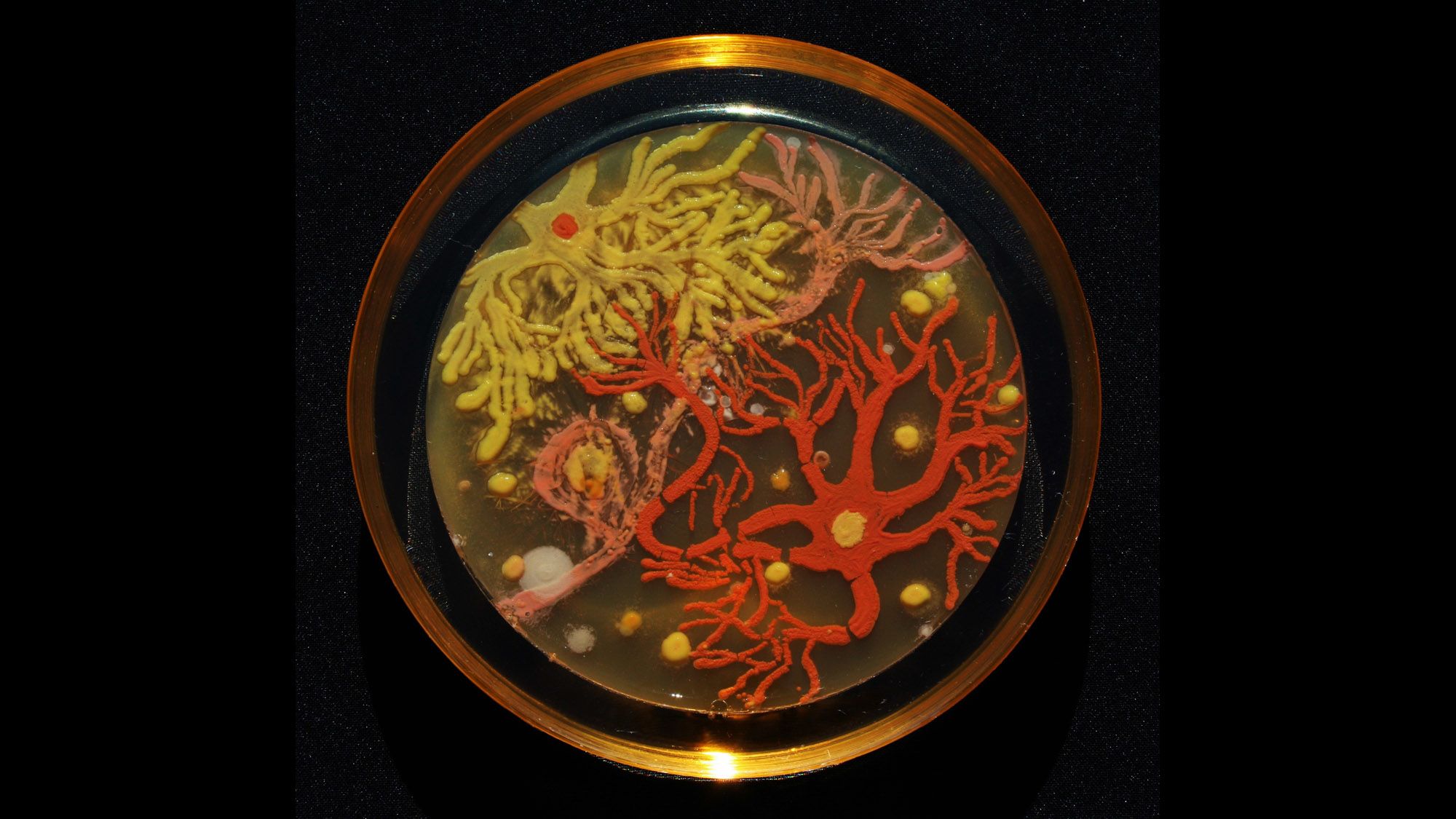The image appears to be a highly detailed close-up of a specimen displayed within a circular petri dish, featuring a distinctive gold or brass outer edge. Set against a stark black background with thick black borders on the sides, the dish contains a complex and vivid arrangement that resembles branching bacterial colonies. Dominant features include a yellow branching structure extending across the left side, a central pink pathway, and a red cell-like body on the right with a central yellow dot. These structures branch out intricately into numerous smaller offshoots. Scattered throughout the dish are numerous small yellow splotches, adding to the complexity. The overall impression is both scientific and artistic, capturing the microscopic beauty and the somewhat disconcerting nature of bacterial growth.